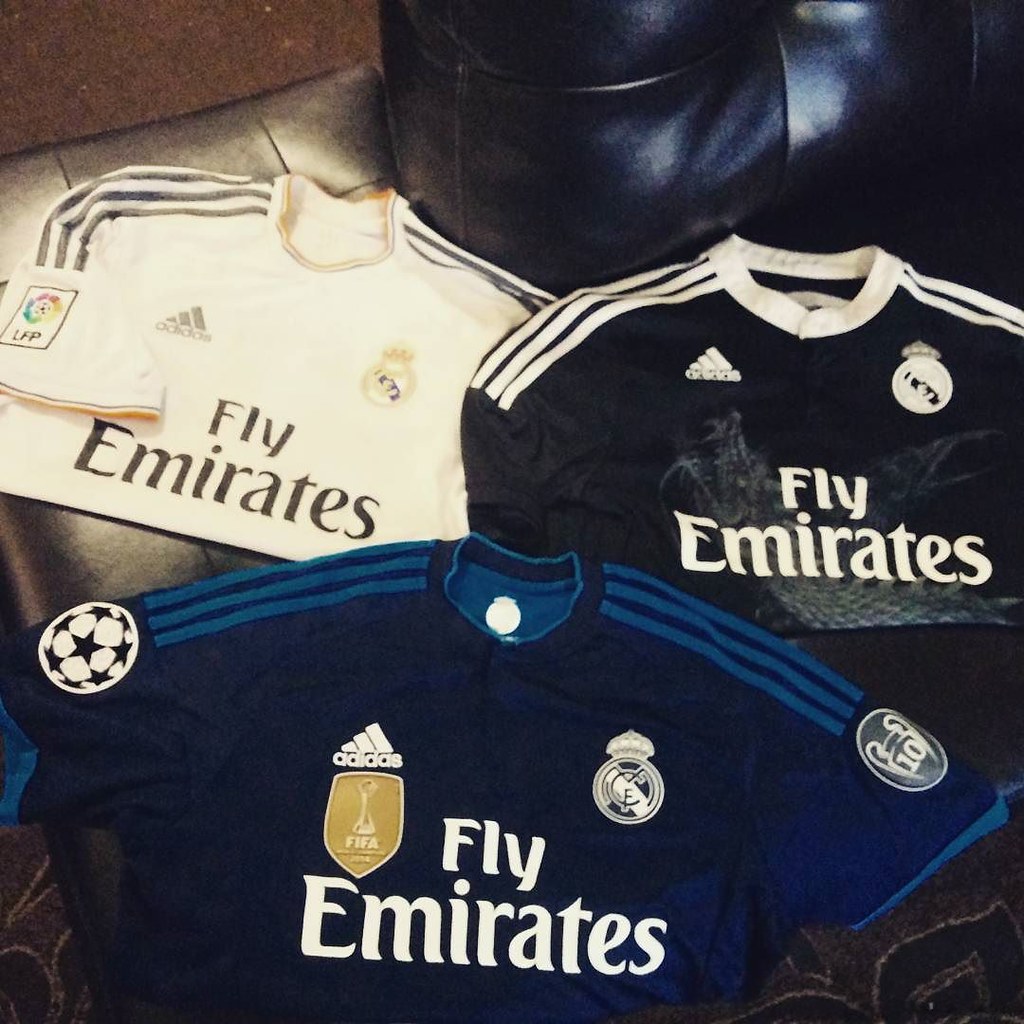This color photograph captures three soccer jerseys arranged on a shiny black leather chair, likely an armchair. The top left jersey, predominantly white with black shoulder stripes, features a rainbow-colored circle on the left sleeve showcasing a soccer ball and "LFP." The right chest bears the Adidas logo, while the left chest displays a crest with a crown. Across the front, "Fly Emirates" is printed in bold black letters. The top right jersey is black with white shoulder stripes and collar, mirroring the Adidas logo on the right chest and a crown crest on the left. Below the text "Fly Emirates," the jersey reveals a subtle gray dragon design. The bottom jersey, navy blue with light blue shoulder stripes, includes a unique patch on the left sleeve depicting a soccer ball with star shapes. The Adidas logo appears on the right chest above a gold FIFA badge, and the front reads "Fly Emirates" in white.